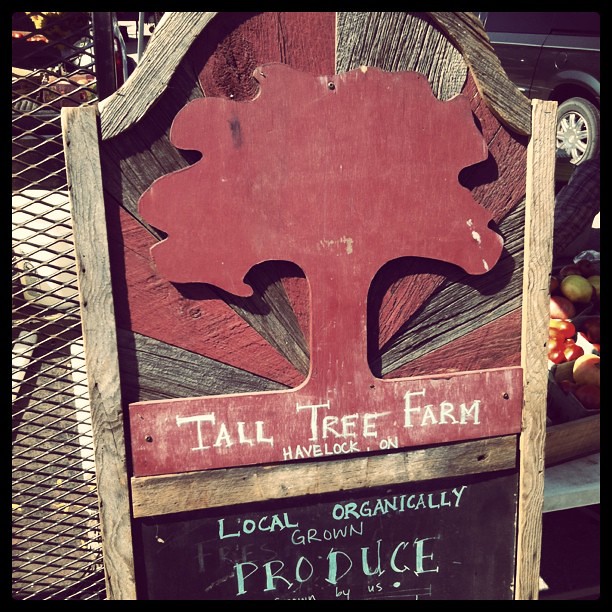The image showcases a detailed and creatively crafted wooden sign for "Tall Tree Farm" located in Havelock, ON. The sign is designed in the shape of a red-painted wooden tree, which stands out prominently against a layered wooden background that blends natural wood tones with additional red paint. The top of the sign features an arch to fit the tree cutout, providing a whimsical touch to the otherwise rectangular design. Below the tree trunk, the business name "Tall Tree Farm" is displayed in a serif font, while "Havelock, ON" appears below in a sans-serif font. Further down, a black section resembling a chalkboard is inscribed with the phrase "Local Organically Grown Produce" in green chalk. The scene behind the sign includes a metal fence, a black car, and an array of colorful fruits, indicating the farm’s offerings. A trailer is visible on the left side of the image, contributing to the farm-like atmosphere.